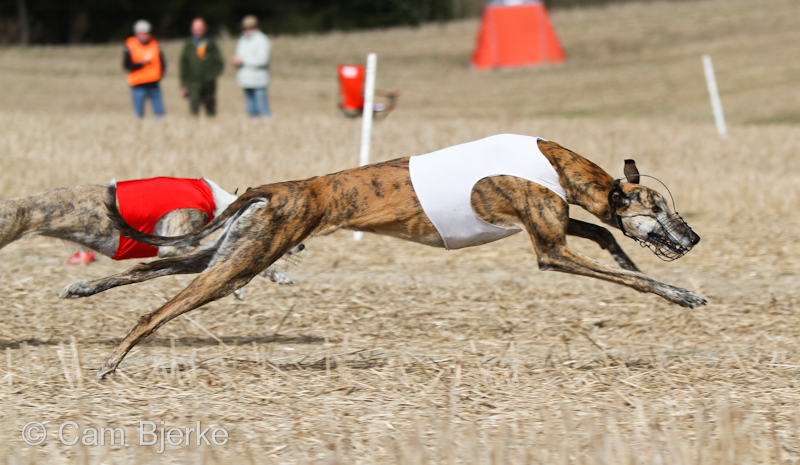In this outdoor scene, the photo captures two greyhounds in the midst of an official race, sprinting across a vast, neutral beige field covered in dry grass. The dogs, with their lean, muscular bodies typical of the breed, are both airborne except for a slight touch of one paw on the ground, demonstrating their impressive speed. The foremost greyhound is outfitted in a white racing vest and sports a metal muzzle around its snout, which is detailed with black elements and cords. The second greyhound, partially obscured behind the first, wears a red vest. In the background, there are three spectators observing the race; one is distinguishable by an orange safety vest, standing near what appears to be a red folding chair and an orange tent. The field and its sparse, dried grass stretch out under an open sky, emphasizing the desolate yet charged atmosphere of the race.